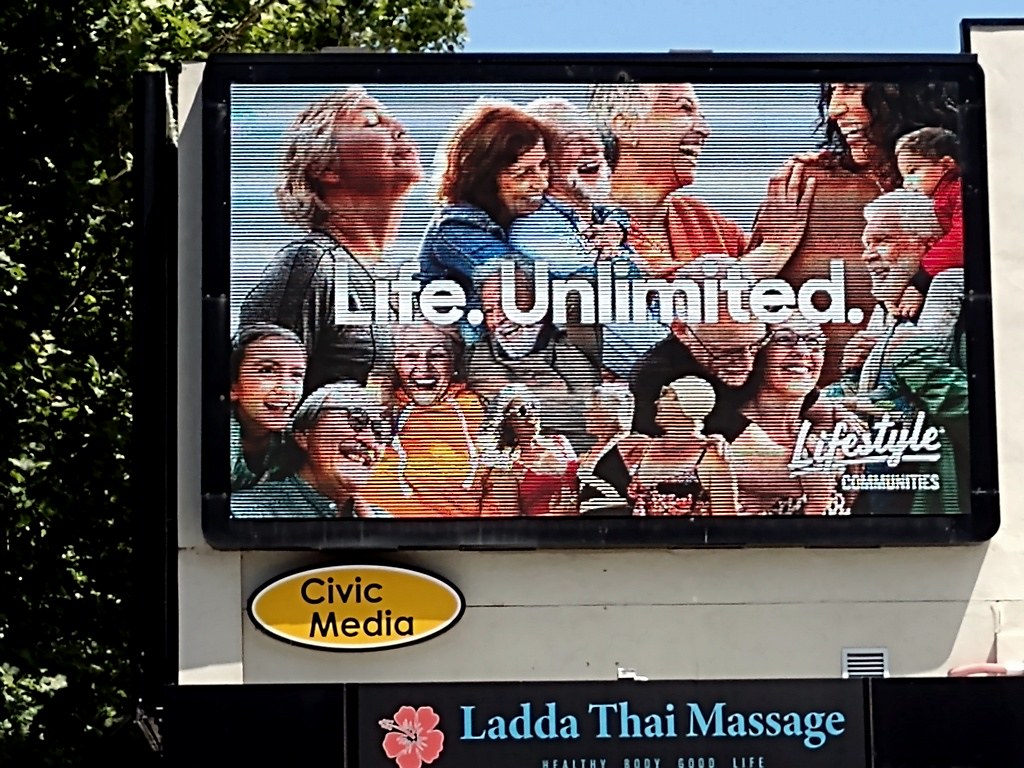You are looking directly at a large billboard set against a clear, light blue sky devoid of clouds. Adjacent to the billboard on the left side is a sprawling, lush green bush. The billboard itself features a white background with a central image framed in black. 

The image showcases several older individuals, predominantly women aged around 40 and above. In the bottom left corner, a young girl gazes over the shoulder of an older woman with a short, banged haircut. In the top right corner, a small child in a red sweater and jeans stands out. Among the figures, another noticeable presence is a man with gray hair and a beard, clad in a gray shirt. Scattered throughout are more elderly women and men.

At the bottom of the billboard, the text reads "Lata Thai Massage."